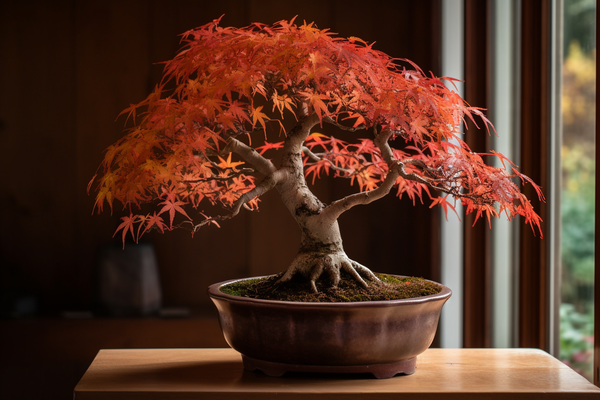A small Japanese-style bonsai tree sits elegantly in a shiny bronze-colored pot, which contains moss-covered dirt. The bonsai, robust and meticulously shaped, features a white bark reminiscent of a white oak or birch. Its intricate root system extends visibly from the soil, giving rise to a beautifully twisted trunk. The tree boasts three substantial branches with numerous smaller ones, all adorned with vibrant foliage ranging from deep red to bright orange. Each leaf is star-shaped, contributing to the tree's striking appearance. This artwork-quality photograph captures the bonsai on a polished wooden table, beside a large window through which sunlight streams, illuminating the scene. In the background, partially blurry, are indistinct pieces of furniture and a hint of lush green and yellow foliage outside, enhancing the serene and natural ambiance.